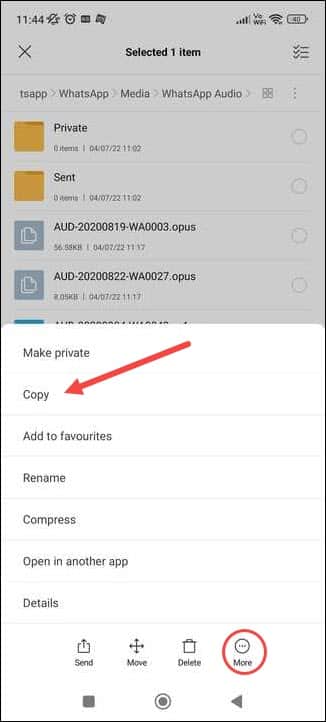The image depicts an Android application running on a phone, identifiable as a non-Samsung device by the standard navigation buttons at the bottom. The background is primarily white with gray navigation buttons: a circular home button in the middle, a square recent apps button on the left, and a left-pointing back arrow on the right.

In the foreground, a contextual menu is open over a dimmed, grayed-out background, enhancing the sense of depth despite the flat design and lack of shading. This menu features a list of options on a white backdrop, with a prominent red arrow pointing to the "Copy" option. Above "Copy," the menu options include "Make private," and below it, the options include "Add to favorites," "Rename," "Compress," "Open in another app," and "Details."

There is also a row of four circular icons with labels underneath. The selected icon, circled in red, is labeled "More" and represented by an ellipsis. To its left, the icons are "Delete" (a trash can symbol), "Move" (arrows pointing in four directions), and "Send" (a send logo).

In the grayed-out background, a file directory structure is visible, suggesting the user is browsing their files. A bold banner at the top indicates that one item is selected, followed by the file path: "WhatsApp > WhatsApp Media > WhatsApp Audio." Within this directory, two subfolders named "private" and "sent" are visible. Additionally, files labeled with "AUD" followed by a string of numbers and ending in ".Opus" are displayed, indicating audio files from WhatsApp.